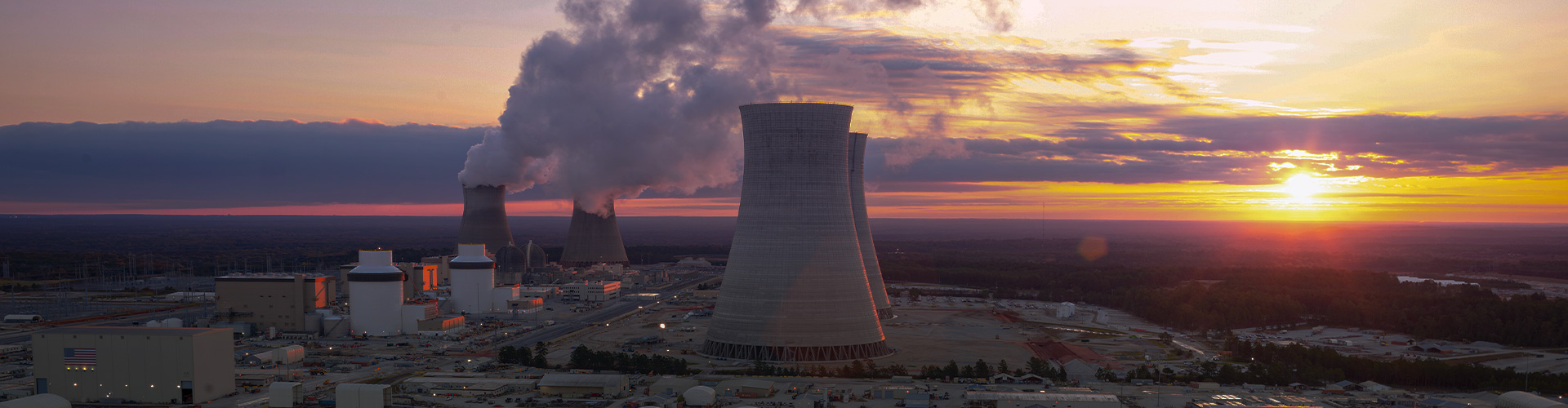The image captures a sweeping view of a nuclear power plant bathed in the warm light of a setting sun. The sky, transitioning through a palette of vivid colors from bright orange to deep purple, is textured with clouds that reflect the fading daylight. Prominent in the foreground are two large, cylindrical towers accompanied by two smaller stacks on the left, all emitting thick streams of steam that blend into the twilight sky. The scene also includes additional smaller buildings at the base of the towers, though they are partially obscured by distance and shadow. A body of water glimmers faintly in the far right corner, suggesting the plant's use of it, potentially for cooling purposes. The surrounding landscape appears to be a mix of countryside and forest, indicating the plant's isolation from urban areas. Overall, the image juxtaposes the industrial might of the power plant against the natural beauty of the sunset, creating a striking and thought-provoking scene.